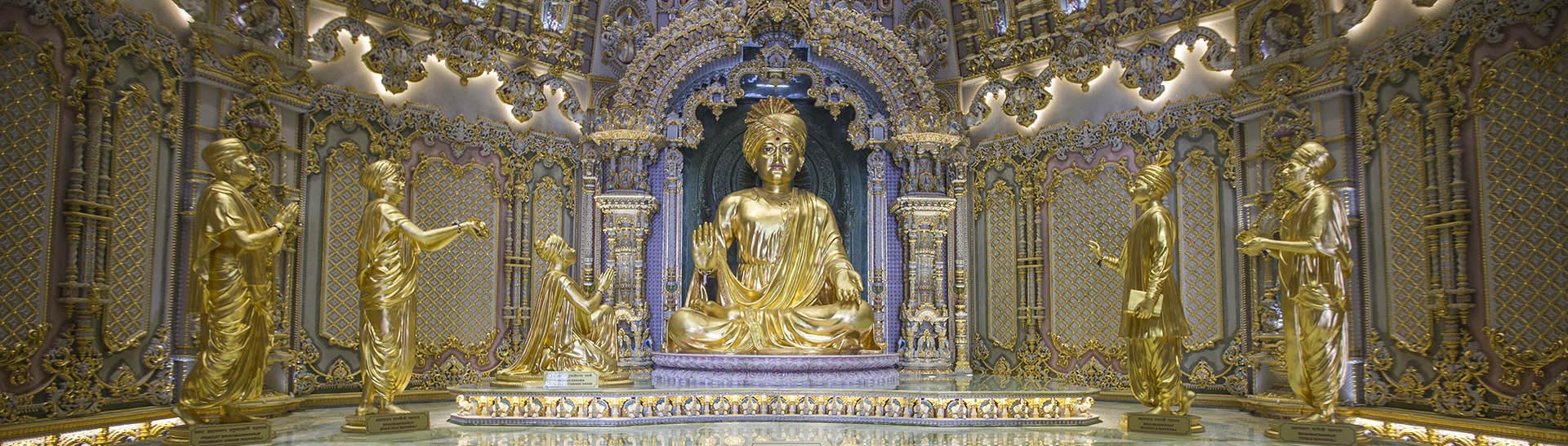The image captures the interior of a lavish Buddhist temple, featuring an arrangement of statues centered around an imposing golden Buddha. The scene is dominated by a large, shiny gold Buddha statue seated in the middle, exuding an air of serene authority. Flanking the Buddha are statues of worshippers, five in total, three on the left and two on the right. These statues appear to be offering gifts and praying, all of which are also adorned in gleaming gold. The Buddha, wearing a golden turban, is ensconced within a shrine that features intricate gold trim and a vivid blue backdrop. The architecture of the building, visible in the background, lends an additional layer of opulence with its white, brown, silver, and clear accents, enhancing the overall grandeur of the setting. The long, rectangular format of the image emphasizes the majestic symmetry and detailed craftsmanship of this sacred space, likely situated in a Buddhist temple in another country.